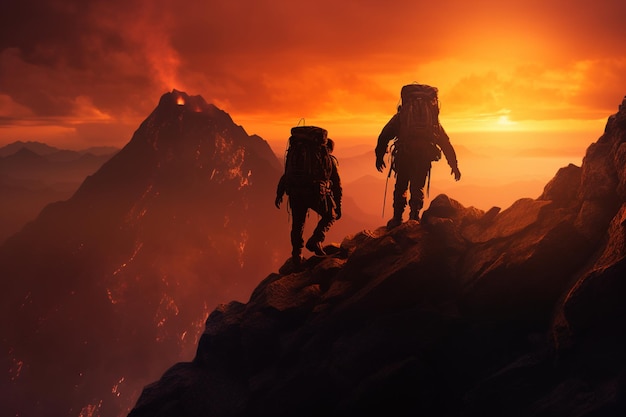In this detailed color illustration, set in a landscape orientation, two determined mountain climbers are depicted ascending a rocky slope near a volcano, amidst a dramatic twilight scene. Positioned near the center, one climber is higher and to the right, facing away from the viewer with his arms outstretched below his waist. He is equipped with a large backpack and other climbing gear secured around his waist. Slightly lower and to the left, the other climber is moving steadily across the rocky terrain, also burdened with a hefty backpack. The sunset casts vivid orange rays, creating a striking contrast against the fiery red smoke emanating from the volcano on the image's left side. This red smoke, darker on the left and gradually turning bright orange towards the setting sun, blankets the upper portion of the illustration. The scene is further enriched by an array of lighter brown mountain ranges in the background, enveloped by scattered clouds, all under a darkened foreground. The emphasis on the climbers, inching forward with each step, encapsulates their relentless determination and the epic nature of their climb.